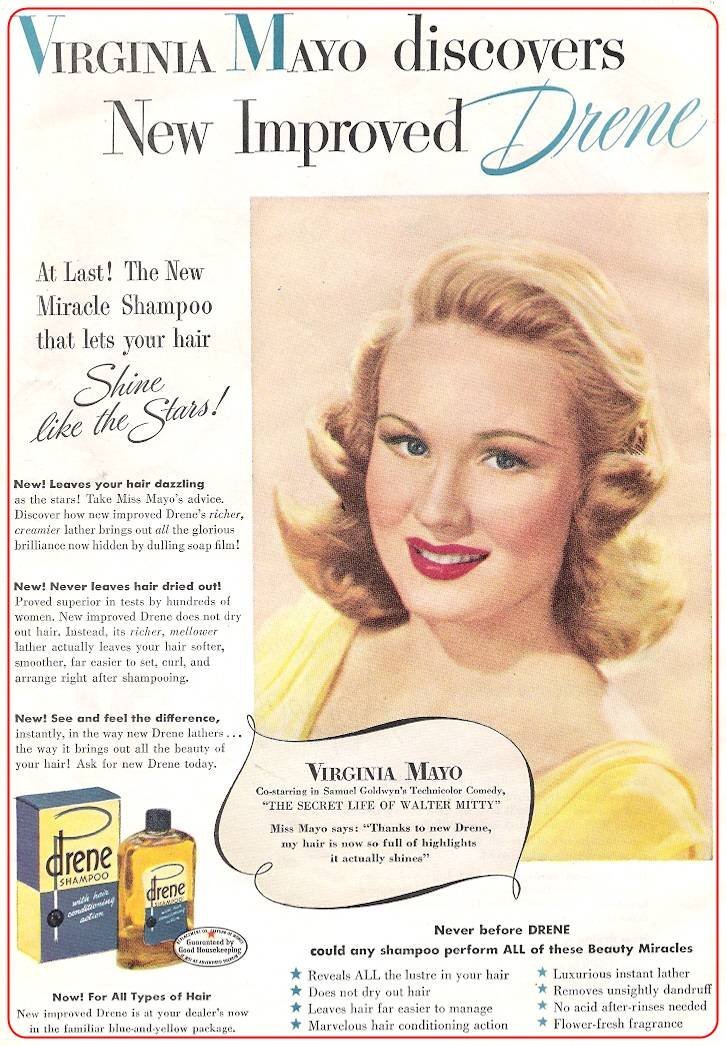This vintage advertisement from the 1940s-1950s features actress Virginia Mayo promoting the newly improved Drene Shampoo. The ad showcases a glamorous blonde woman with red lipstick and a radiant smile, dressed in a yellow outfit. The headline reads, "Virginia Mayo Discovers New Improved Drene." The tagline emphasizes, “At last, the new miracle shampoo that lets your hair shine like the stars,” highlighting the product's benefits such as making hair dazzling, preventing dryness, and offering visible and tangible improvements. The ad includes an image of the shampoo bottle and its packaging, which is displayed on the bottom left. The box is blue and yellow and bears the Good Housekeeping Seal of Approval. The overall design and text-heavy layout evoke the mid-century advertising style, reinforcing the product’s promises of beauty and improved hair care.